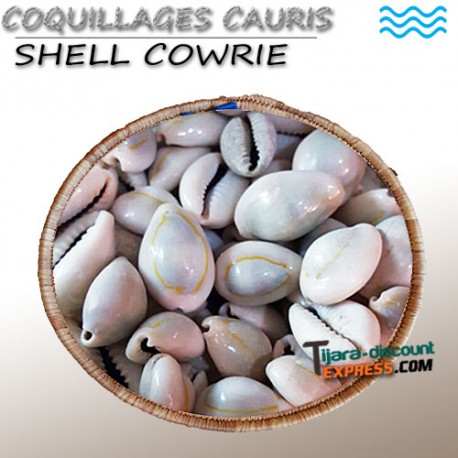Set against a beige background that transitions into a darker tan hue as it moves downward, this image prominently features the text "C-O-Q-U-I-L-L-A-G-E-S, C-A-U-R-I-S" in a textured, gray bold font in the upper left-hand corner. Below this text, there is a horizontal black line, under which "Shell Calvary" is written in black letters with a shadowed effect. The upper right-hand corner of the image displays three wavy blue lines symbolizing waves. Centrally placed is an oval or circular area with a woven circular edge, containing a large pile of white shells resembling mouth-like or lobster claw shapes, some outlined with a delicate yellow line. In the lower right-hand corner, the text "tiara-discount-express.com" appears. The "T" is large and black, "tiara" and "discount" are in green, and "Express" is in bold orange letters with a black shadowed background, followed by ".com" in black.